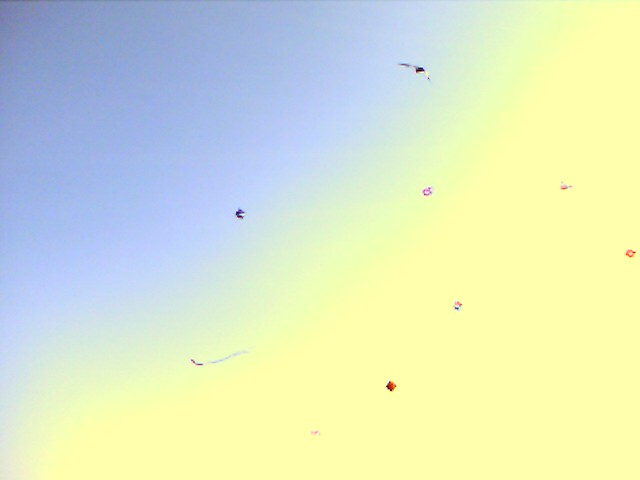A color photograph captures multiple kites soaring high in the sky, seen from the ground below. The sky exhibits a gradient, transitioning from a clear blue on the top left to a greenish hue in the middle, and finally blending into a yellowish tint at the bottom. The image quality is somewhat grainy and fuzzy, making the kites appear as tiny, colorful shapes. Some kites are designed with tails while others resemble small diamond shapes. Notably, one kite mimics the image of a bird with wings spread wide. The kites are predominantly pink, blue, and red, though their precise shapes and details are difficult to discern due to their altitude and the image's clarity.